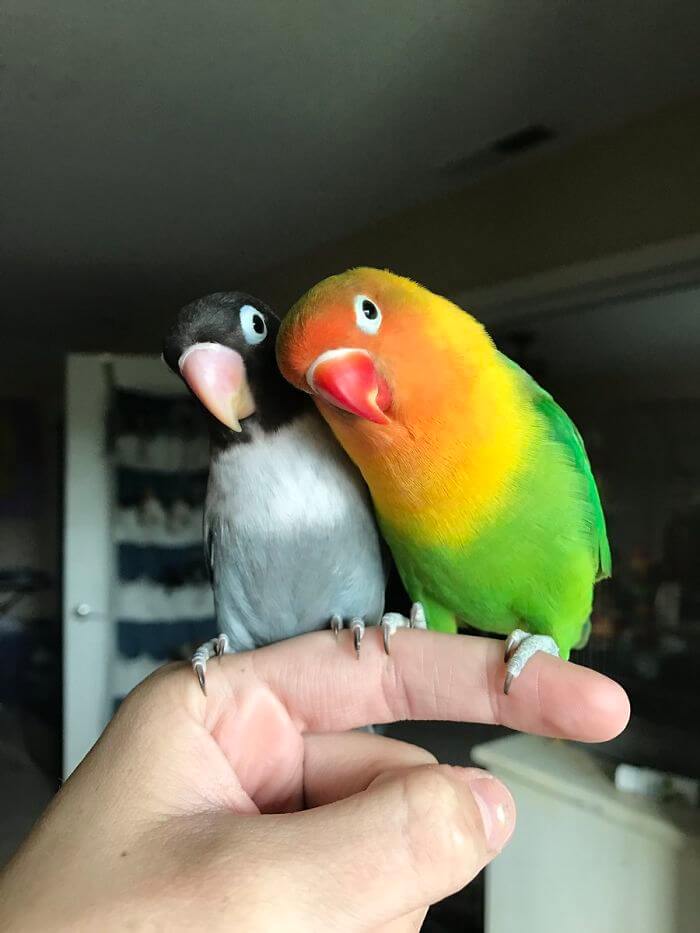In the image, a young man extends his pointer finger, holding the rest of his hand in a fist. Perched on his finger are two small birds, each with its claws wrapped around his finger. The bird on the right is a vibrant lovebird with a striking color gradient: a red beak, a burnt sienna head that transitions into orange around the neck, then yellow, and finally, a bright green body. This bird is tilting its head slightly, showcasing its big, curious eyes. Beside it, the bird on the left contrasts with a black head, a beige beak, a white and gray chest, and white feathers merging into the gray. Both birds lean their heads to the left, appearing inquisitive. The background features a white stand and a door with a shoe rack and a silver doorknob, suggesting the scene is set in a bedroom.